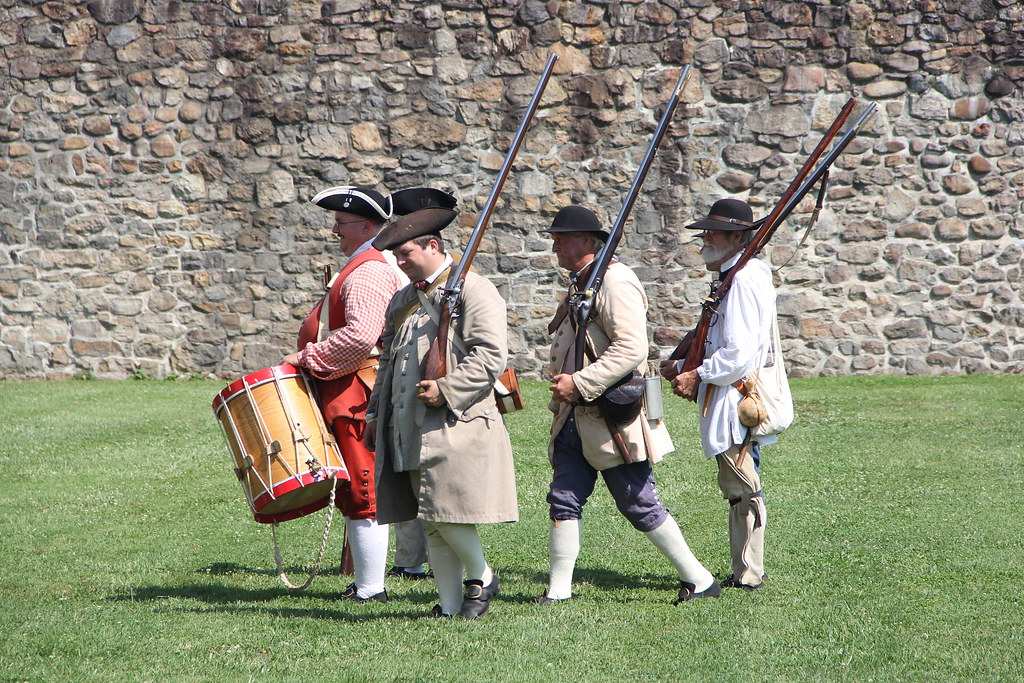In this color photograph taken outdoors during the daytime, four men dressed in historical wartime clothing are standing on a green lawn against the backdrop of a massive old-style stone wall. The man in the center front is dressed in a striking red outfit with a striped red and white shirt, long white socks, and black shoes; he is playing a wooden drum with red edges. He is also wearing glasses. The other three men, also wearing glasses, are dressed in similar traditional attire, including oversized jackets, beige or gray knicker pants, white stockings, and black shoes. They all wear black hats, but each has a slightly different style. These three men are carrying long-barreled rifles or muskets, adding to the reenactment-like atmosphere of the scene. One of the men has a gourd on his waist, and another has a black waist belt bag. They all appear to be walking in the same direction, evoking the feel of a Revolutionary War-era procession.